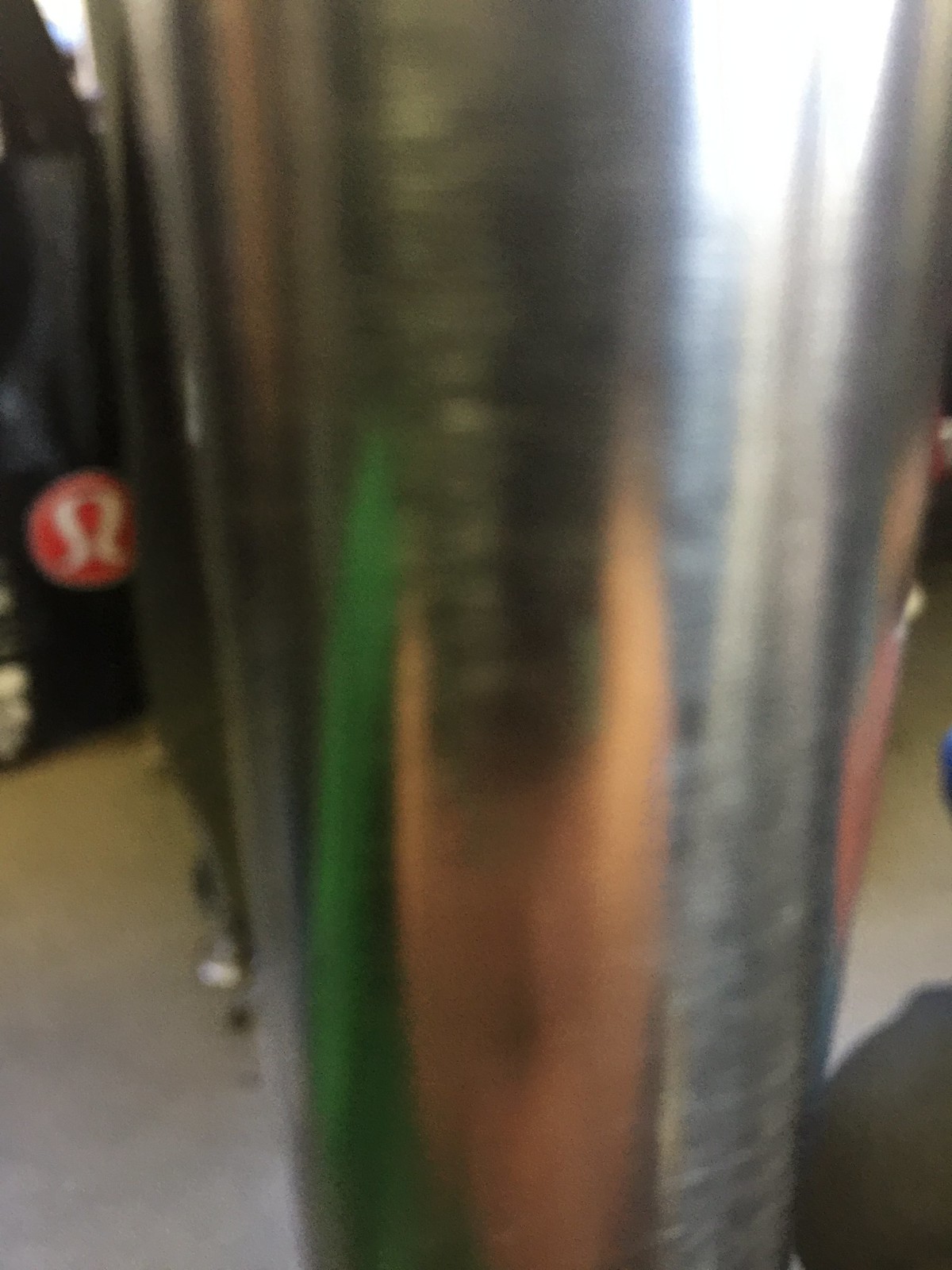Despite the extreme blurriness of the image, the setting appears to be outdoors, possibly featuring a sidewalk in the background. Shadows cast upon the sidewalk suggest the presence of individuals. A highly reflective silver pole is prominently visible, capturing the reflection of a likely male figure. The person in the reflection seems to be wearing a green garment that is open to reveal a bare chest. Additionally, the individual appears to be donning a mask akin to a gas mask, creating an unusual juxtaposition. Another pole can be seen behind the person, leading to speculation whether the image portrays one reflective pole or two distinct poles, with the blurriness causing ambiguity.